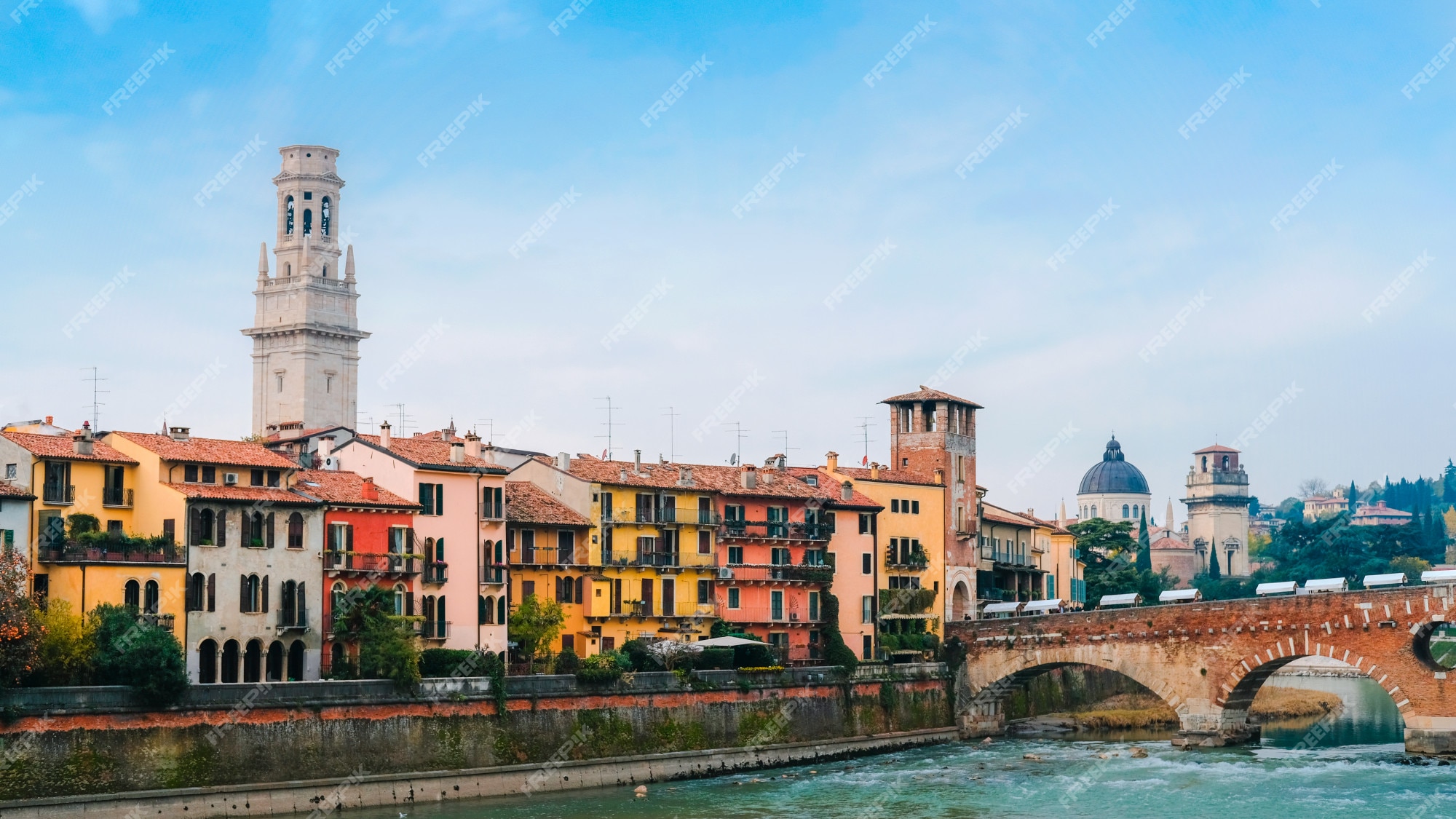This color photograph, taken in landscape orientation, showcases a picturesque riverside town with a vibrant array of high-rise buildings in various pastel hues such as green, yellow, white, red, and pink. The town lies along the Adige River in Verona, Italy. The image captures a broad blue sky adorned with white clouds, and sunlight brightens the scene, emphasizing the town's colorful architecture. 

At the center-right of the image, an arched bridge, constructed from distinctive red bricks with a stucco application, spans the river. The bridge features openings underneath to allow boats to pass through. Adjacent to the river, there's a raised wall, weathered and covered in moss, with a red-bordered fence atop it. This wall likely serves as a flood barrier. 

Buildings line the riverfront, displaying architectural diversity with towering spires, dome-shaped structures, and traditional facades. Notably, a white tower stands out behind the multicolored buildings on the left, and a gray domed structure is visible in the distance on the right. The river, with its murky green water, appears widest at the bottom of the image and recedes into the background to the right, adding depth to the photograph. The entire image is marked with a white diagonal watermark reading "Free Pix."